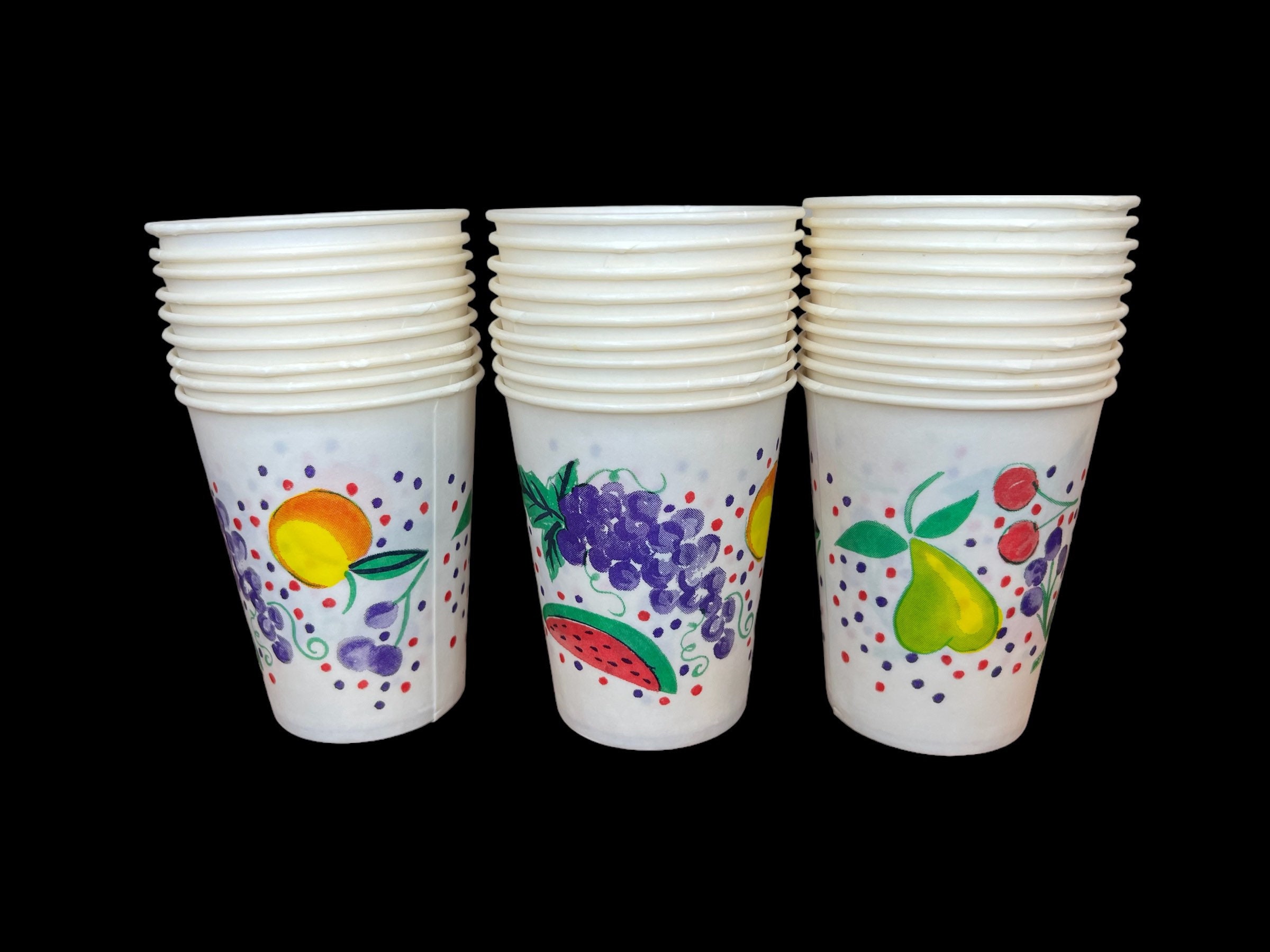The photograph features three neatly stacked columns of ten white paper cups, each adorned with festive, fruity patterns. Against a black backdrop, the cups present a vibrant parade of cartoonish fruit designs and colorful polka dots. Displayed upright as if ready for use, the first stack showcases an orange surrounded by red and purple polka dots, alongside a glimpse of cherries and a cluster of grapes. The middle stack, turned slightly to reveal more of the pattern, prominently features a cluster of purple grapes and a juicy slice of watermelon, continuing the playful polka dot motif. Finally, the stack on the right reveals a detailed depiction of a greenish-yellow pear with leaves, accompanied by cherries and a few additional grapes, completing the cheerful and eye-catching design.